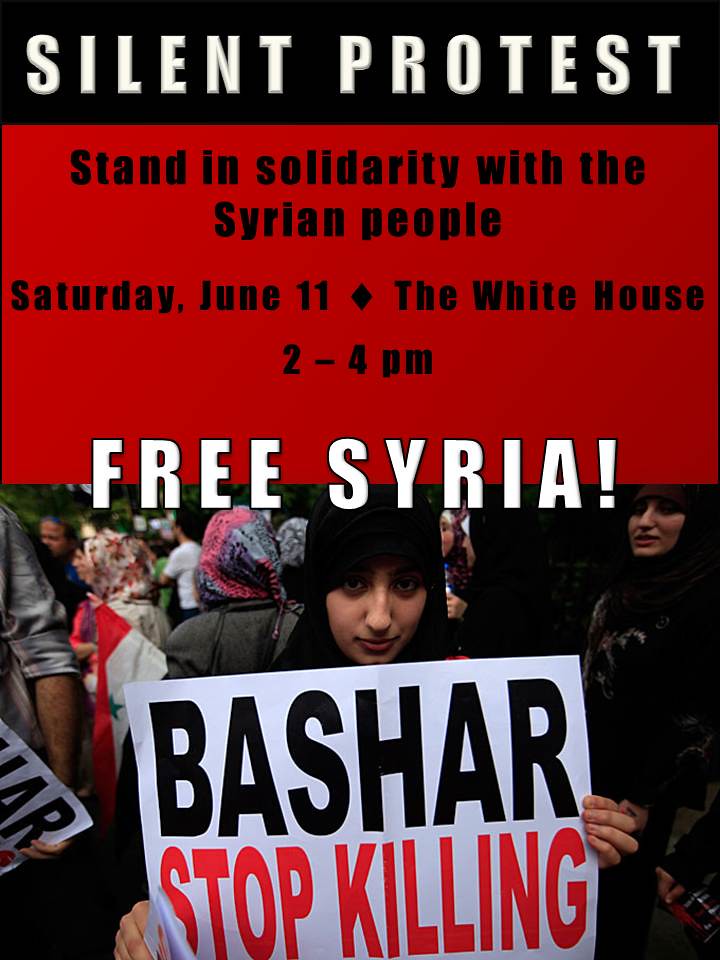This tall rectangular image is a powerful poster advocating a silent protest in support of Syria. At the top, a thick black bar stretches across with large white, all capital letters reading "SILENT PROTEST." Below this, a thick red rectangle boldly announces in black text, "Stand in Solidarity with the Syrian People, Saturday, June 11th, The White House, 2 to 4 p.m." Directly beneath, in bold white all capital letters, the message "FREE SYRIA!" stands out with an exclamation point. 

A striking photograph captures a woman at the core of the image, draped in a black hijab, situated in a crowd. She holds a wide white rectangular sign that poignantly reads "Bashar" in black at the top and "Stop Killing" in red at the bottom. Around her, numerous individuals stand in solidarity, some holding flags with red, white, and black stripes adorned with a green star, emphasizing the Syrian flag. The crowd also includes people with various headgears and outfits, highlighting the diverse support for the cause. This vivid depiction underscores the ongoing violence in Syria under dictator Bashar al-Assad and the global demand for peace and freedom for the Syrian people.